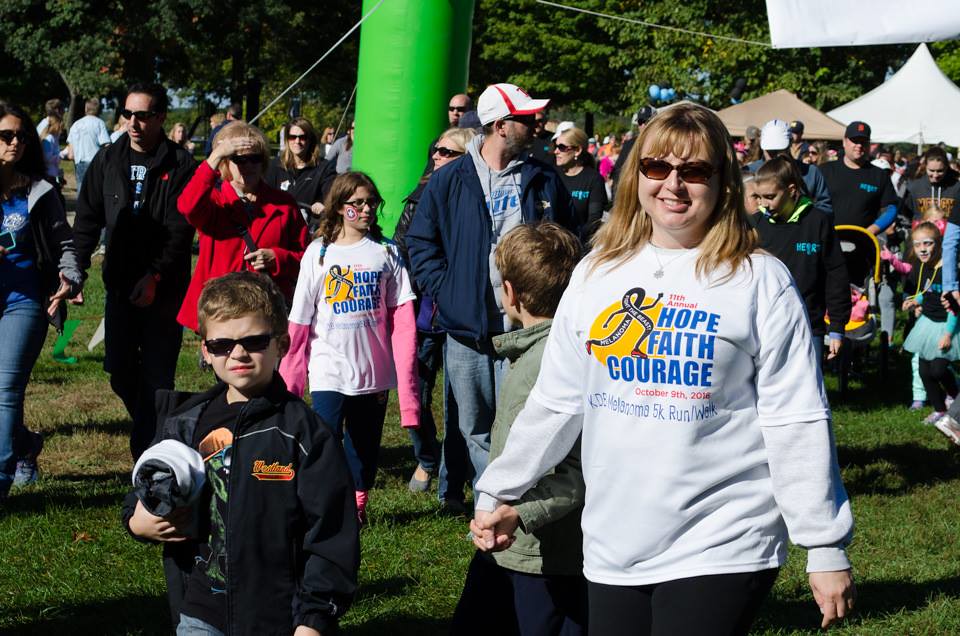The photograph captures a lively, colorful outdoor event, likely a faith-based fair or a melanoma 5K walk for cancer research, set in a grassy area surrounded by trees. Dominating the center of the image is a tall, bright green pole. To the right side, several tents (easy-up canopies) dot the scene, providing shade and gathering spots for attendees. Crowds of people are dispersed throughout, with many facing the camera, appearing to prepare for or engaging in the walk.

In the foreground, a woman in her mid-30s stands out. She has shoulder-length blond hair, wears sunglasses, and is beaming a smile straight at the viewer. She is dressed in a long-sleeved white sweatshirt that reads "Hope, Faith, Courage" in blue letters with a yellow circle featuring stylized running legs. She is holding the hand of a young blond boy who is facing away, wearing a jacket. To her left, another young boy, around 10 years old, sports dark sunglasses and a black jacket, clutching something in his hand.

Further back, a girl in a pink sweatshirt and glasses can be seen. She also wears a white T-shirt with the same "Hope, Faith, Courage" graphic. The event appears to be taking place in the late afternoon with long shadows cast on the ground, and many attendees, including a woman in red shielding her eyes with her hand, are wearing sunglasses against the bright sunlight.